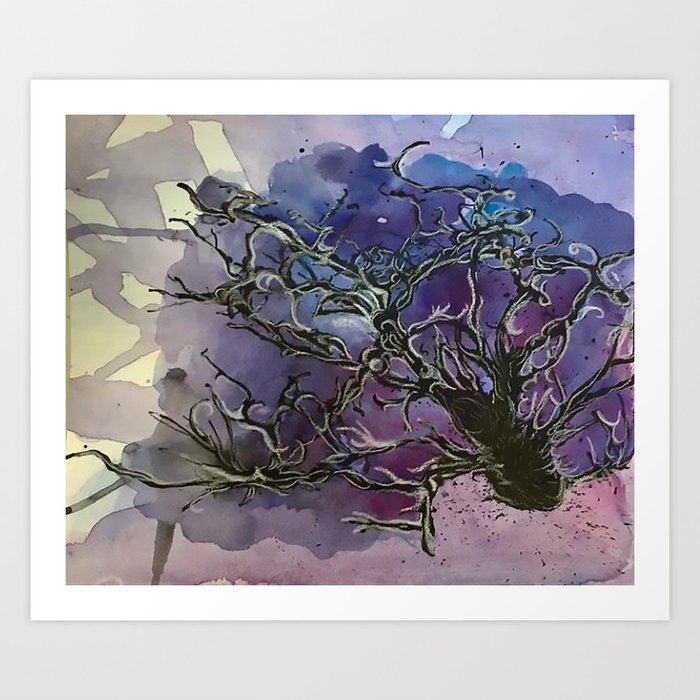The image is a square watercolor painting of approximately 6 inches by 6 inches, surrounded by a matting with a light gray border about half an inch wide at the top and bottom, and a thin white border roughly a quarter of an inch wide. The painting features an abstract composition dominated by shades of purple, blue, and black, with touches of gray and white.

In the bottom right corner, a round, black object is depicted, which could be interpreted as a root or a large insect due to its vein-like strands branching out diagonally across the image. These black strands extend and curl through the central area of the painting, creating a dynamic, tree-like or plant-like structure without resembling any specific flora.

The background of the painting transitions from a very light purple, almost cloud-like at the bottom, to deeper purples and blues with white highlights. To the left, the background shifts to a faint cream color with more geometric shapes in light purple, creating a contrasting backdrop to the organic, free-form strands. Swirls and splatters of purple paint add to the abstract nature of the artwork, enhancing its complexity and ethereal quality.